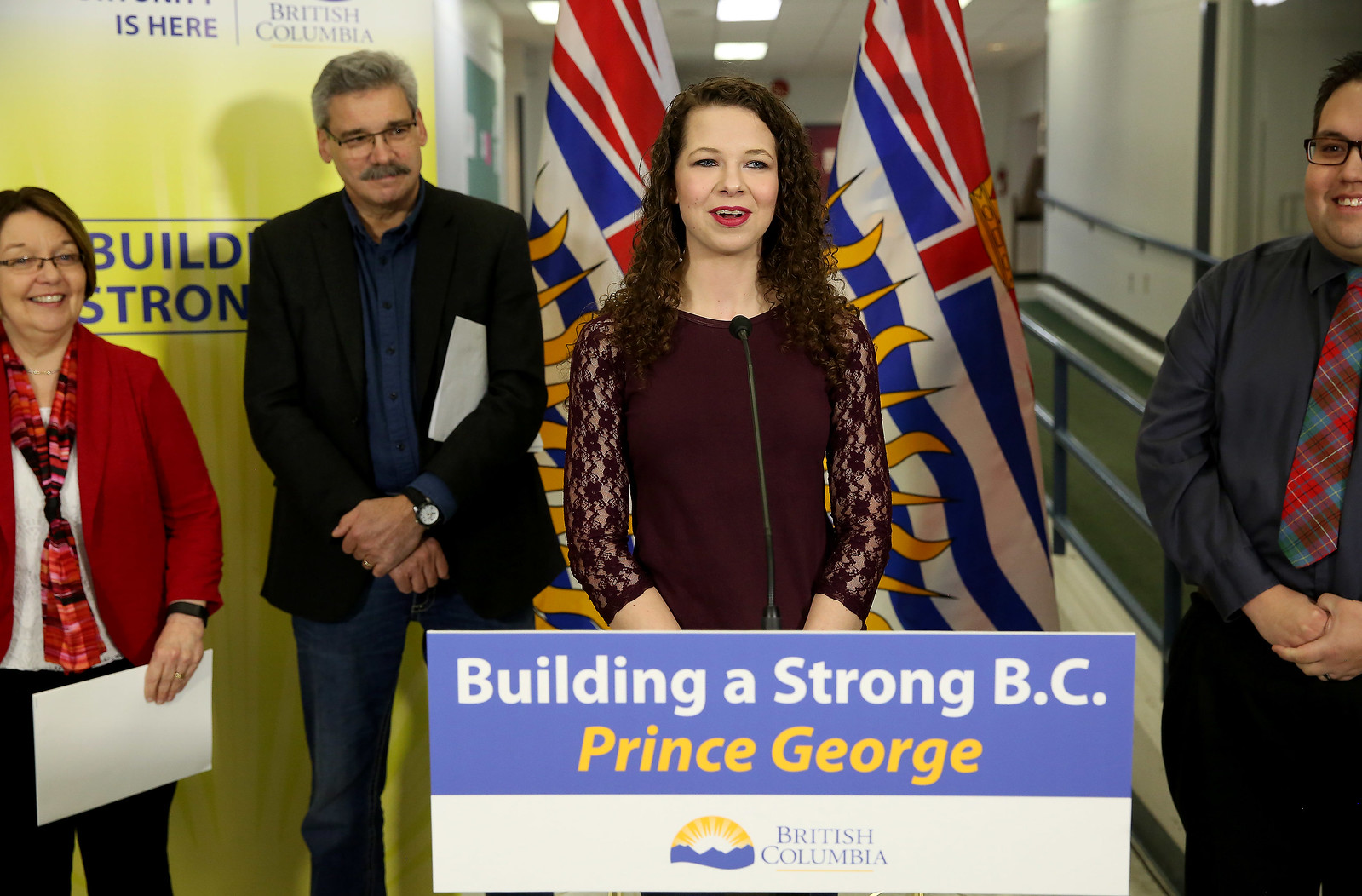The photograph depicts a woman with short, dark brown hair and red lipstick standing at a podium, speaking. She is wearing a wine-colored red dress with long lace sleeves that go just past her elbows. The podium has signage that reads "Building a Strong BC, British Columbia, Prince George," with a British Columbia symbol underneath. Behind her are three other people. To her right stands a man with short black hair, black glasses, a black dress shirt, black pants, and a red and green plaid tie. On her left are a man and a woman. The man is wearing jeans with a blazer and glasses, holding a clipboard under his arm. The woman, partly out of the frame, is in business attire with a blazer and a scarf. Flags of British Columbia are visible behind them, and there's a hallway in the background with visible lighting. The scene appears to be set in an office building, and all attendees are smiling and focusing on the woman at the podium.